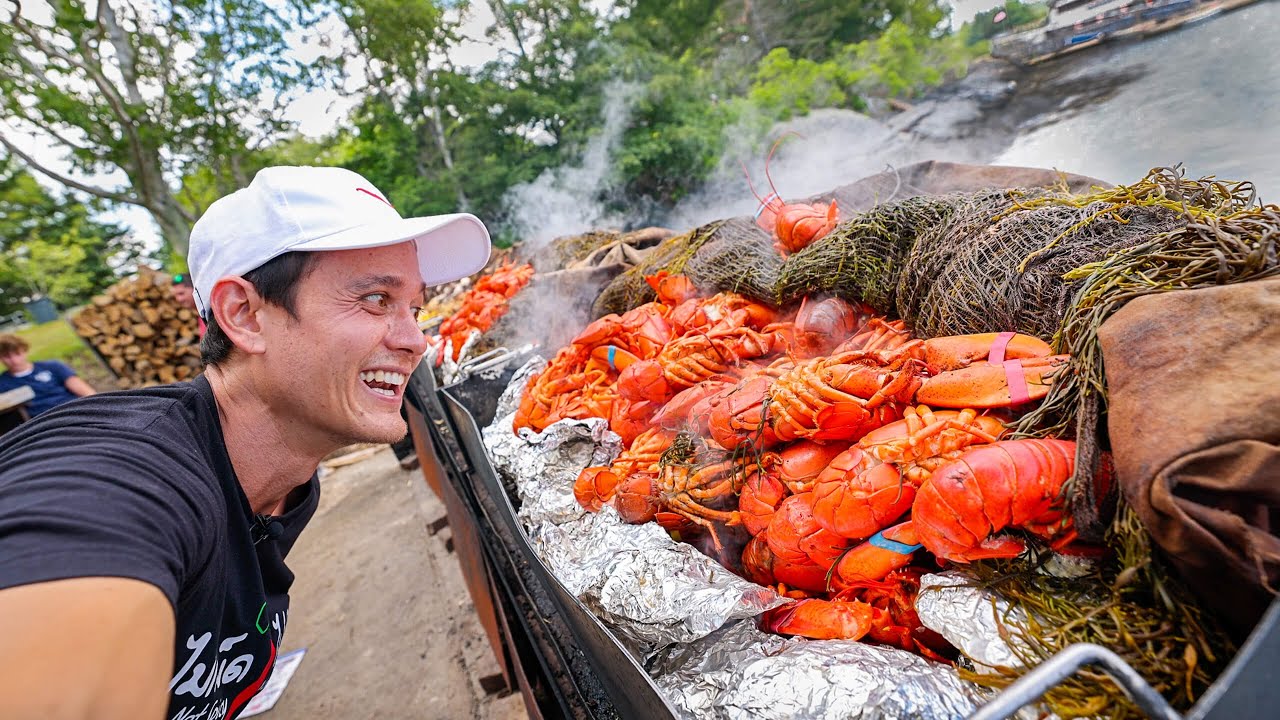The image captures an outdoor scene in a park or waterfront setting, featuring a man standing prominently next to a large silver tray filled with bright orange, steaming lobsters and aluminum foil. He is wearing a white hat with a black logo, has short black hair, and dons a dark navy blue shirt with white text, possibly in South Asian script. The man is smiling broadly, looking at the lobsters with an apparent sense of excitement and pride, and holding the camera with his right arm for a selfie-like shot. Behind him stands a blonde-haired boy in a blue shirt with a white label, expressionless and close to a substantial pile of chopped firewood. To the right, a body of water is visible, suggesting the source of the fresh seafood. The scene is vibrant and lively with additional details such as a fishing net, a green bag, and scattered seaweed around the tray, further emphasizing the narrative of a joyful seafood catch and cook-off event.